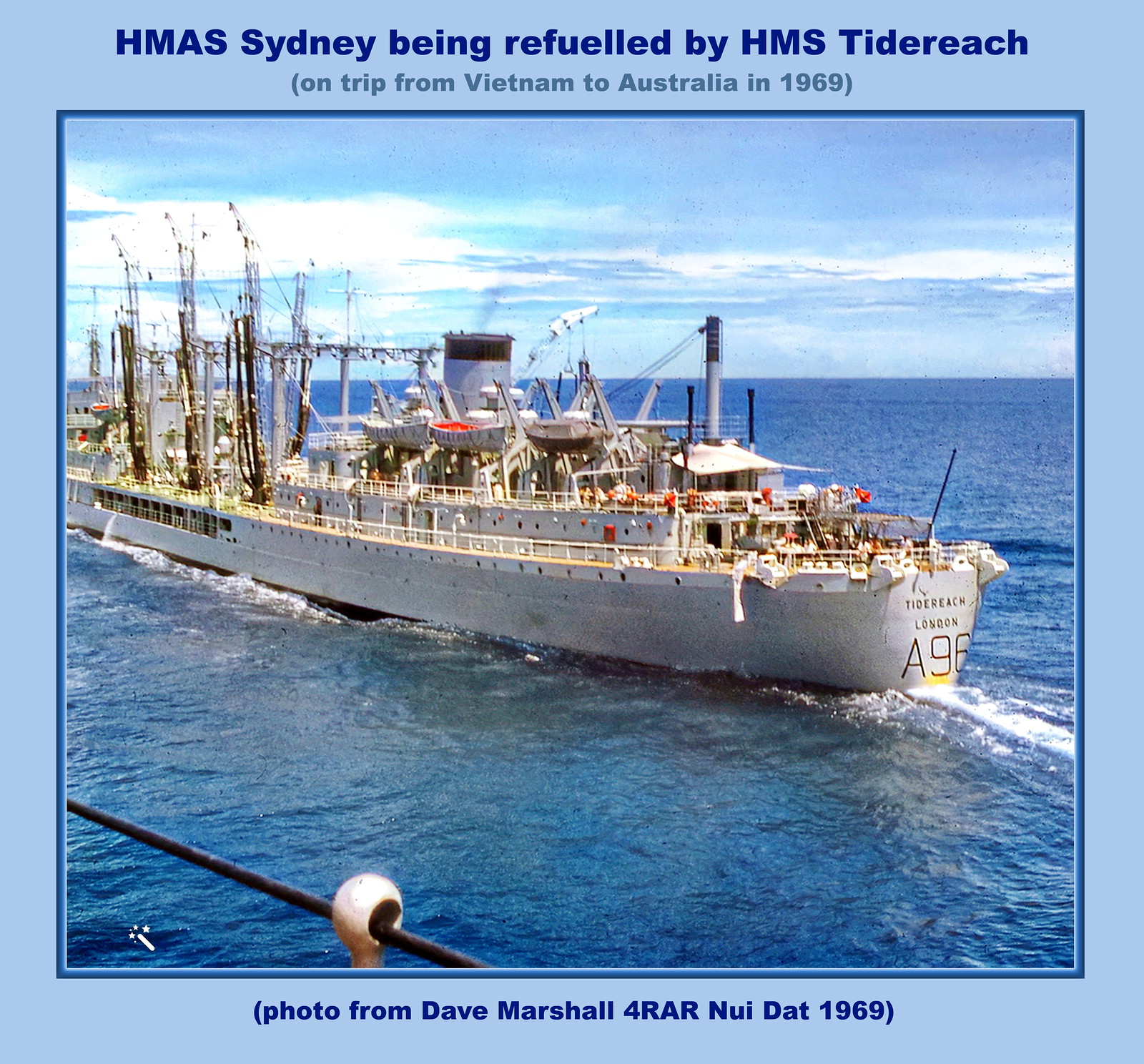This is a color photograph with a narrow blue border and blue text at the top that reads, "HMAS Sydney being refueled by HMS Tide Reach." The image captures a large ship, identified as HMAS Sydney, in the middle of a blue ocean with a clear sky and clouds in the background. The ship features lifeboats hanging on its sides, a prominent smokestack, and crane-like arms. In the foreground, on the lower left-hand side, there is the railing of another vessel from which the photo is taken. The stern of HMAS Sydney displays the text "Tide Reach London A 96." Beneath the main caption, smaller blue text notes, "On trip from Vietnam to Australia in 1969." A white border at the bottom of the image carries the credit: "Photo from Dave Marshall for RAR NUI DAT 1969."